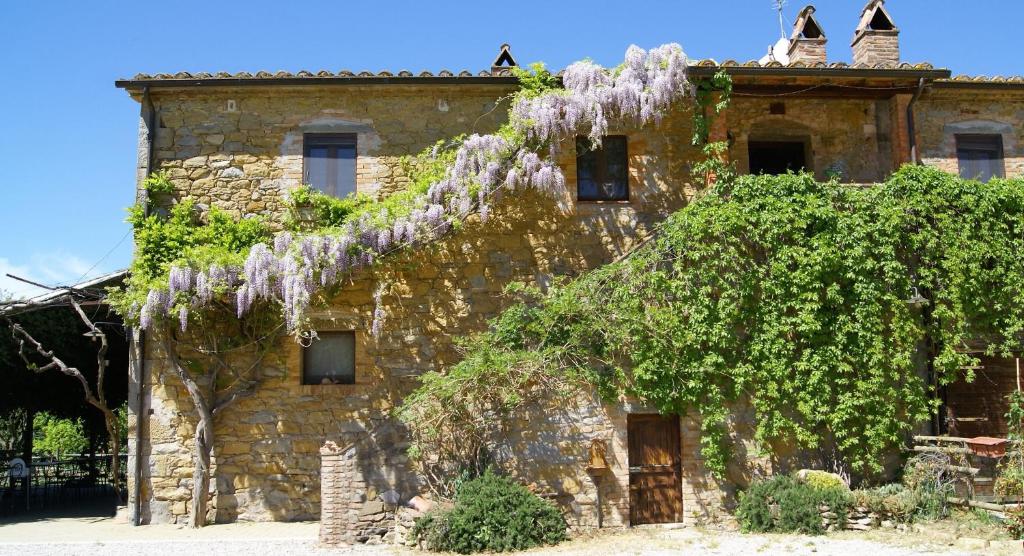In this photo, a picturesque Mediterranean-style adobe stone house dominates the scene. The three-story residence, constructed of tan and gray patchwork stones, features three distinguishing turrets on the upper levels. A covered stairway ascends to the third story, where a wooden door is prominently centered. The exterior walls are adorned with lush greenery, including vibrant grapevines creeping from the left-hand side of the house towards the center, producing clusters of purple flowers that hang elegantly. The slate roof with half-round tiles adds to the home's rustic charm, complemented by five small, square, old-fashioned windows and two chimneys. A dark, covered area, potentially a shed or patio, is positioned to the far left with vines growing beneath it. The yard is devoid of grass, enhancing the house's desert-like, yet inviting ambience under a bright blue sky with minimal clouds.